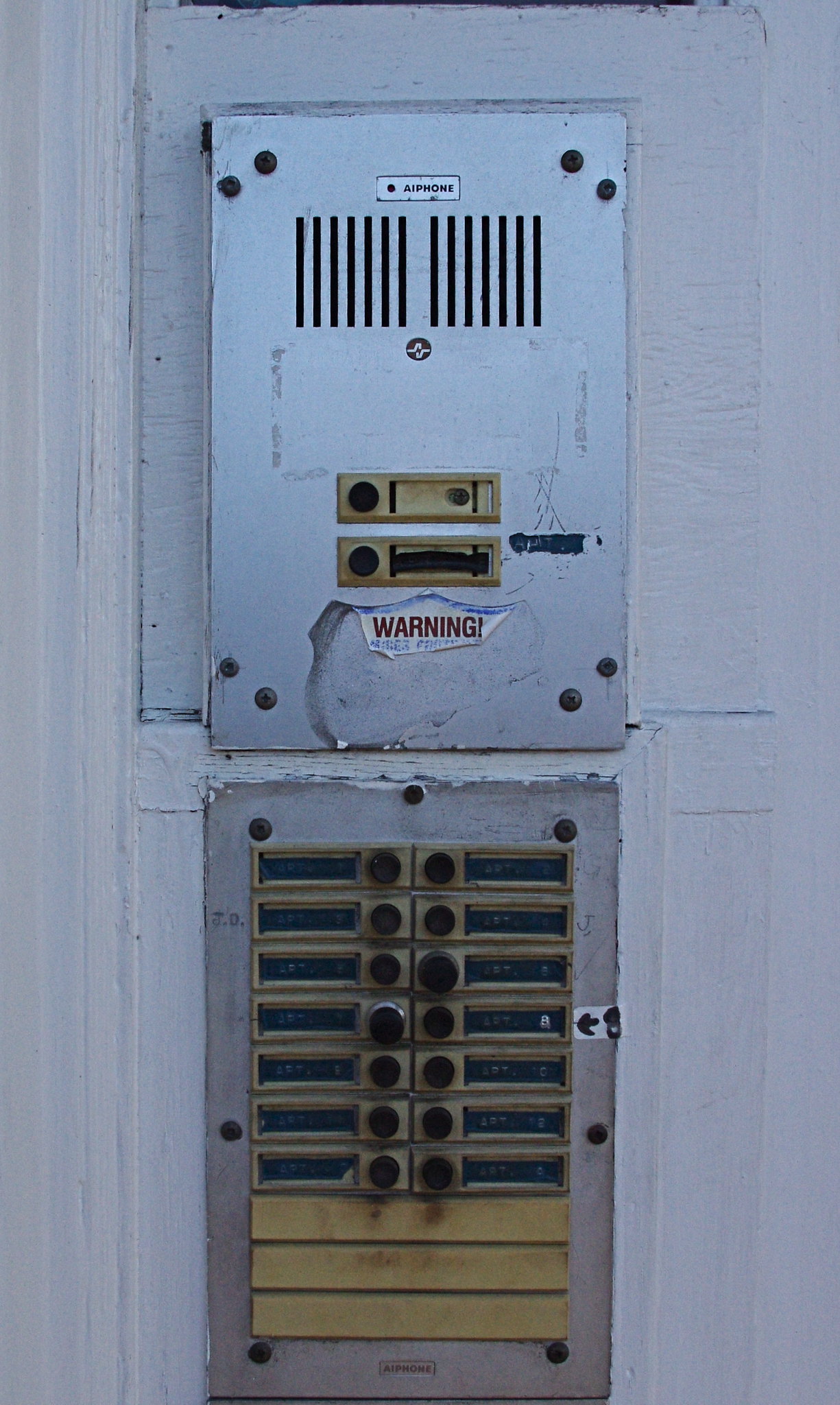The image depicts a detailed close-up of an older building's door entry system mounted on a white wall. At the top, there is a metal intercom panel made of off-white aluminum, featuring speaker slits for voice communication. This panel is secured with eight screws and holds a red warning sticker against a white background, though the sticker is partially peeled off. Below the intercom, there is a second metal panel, also off-white and bolted with seven screws. This bottom panel contains an array of buttons structured in two rows of two buttons each, flanked by small rectangular sections that presumably once displayed apartment names, although these are now blank. Further down, three horizontal yellow bars span the width of the panel, possibly intended for labeling. The entire entry system, both panels, and their various components are all clearly visible in a brightly lit setting.